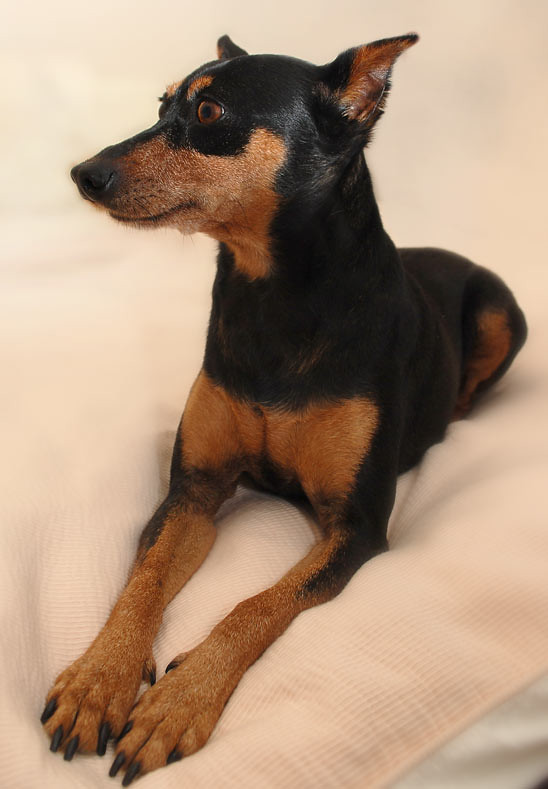In this image, a young Doberman, with a sleek black and tan coat, lies alertly on a lightly colored, ribbed comforter. The bedspread, an off-white or beige hue, appears subtly indented under the dog's weight, accentuating its comfortable yet vigilant pose. The Doberman's ears are drawn back and pointed, highlighting its attentive demeanor as it gazes to the left, relative to the viewer. Its expressive brown eyes, with pupils encased in a faint red outline, peer intently, while its pointy snout adds to its alert expression. Both front paws, adorned with black claws, are extended forward on the fabric, while its tucked hind legs suggest a relaxed position. The lighting softly illuminates the dog from above, casting gentle shadows beneath. The background is blurred, ensuring that the focus remains solely on the poised and watchful puppy.